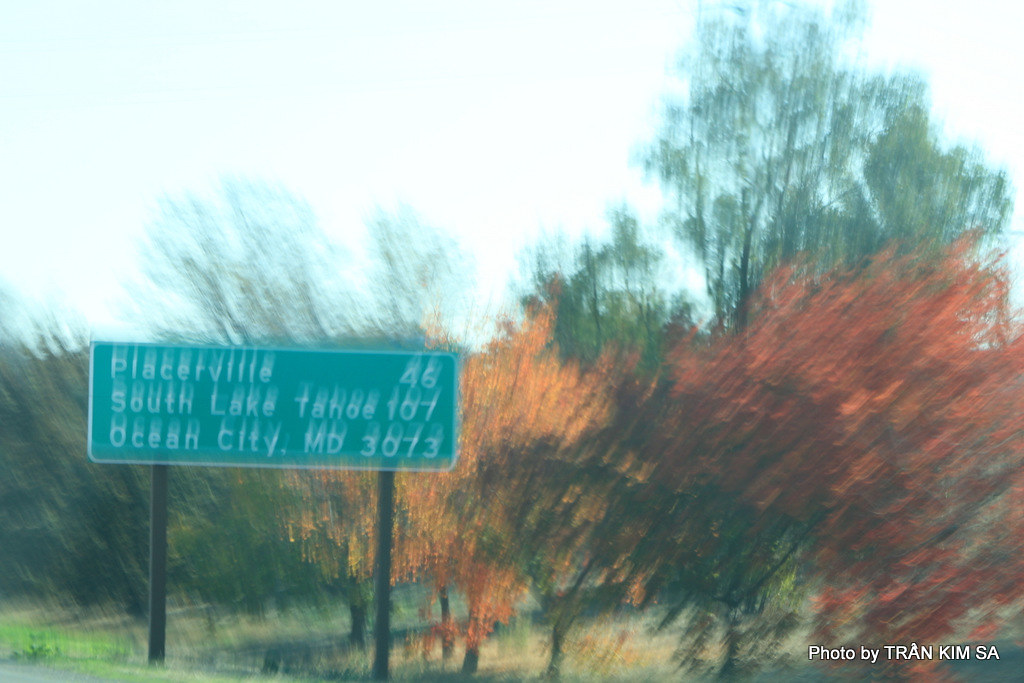The photograph captures a vibrant fall landscape, taken from inside a moving vehicle, evidenced by its slight blurriness. Dominating the scene is a green rectangular highway sign with white lettering mounted on two brown wooden poles. The sign, partially obscured by motion blur, reads: "Placerville 46," "South Lake Tahoe 107," and "Ocean City MD 3073 miles." Beneath the sign, set against a backdrop of autumn foliage, the trees showcase a vivid spectrum of colors—deep reds, bright oranges, and verdant greens. One prominent tree has nearly lost all its leaves, while others persist in their autumnal hues. The grass below appears brown and lifeless. Overhead, the sky is a mix of cloudy and blue. In the lower right corner, the image bears the inscription "photo by Tran Kim Sa" in white. To the left of the sign, the edge of the roadway is visible, grounding this picturesque scene in its rural setting.